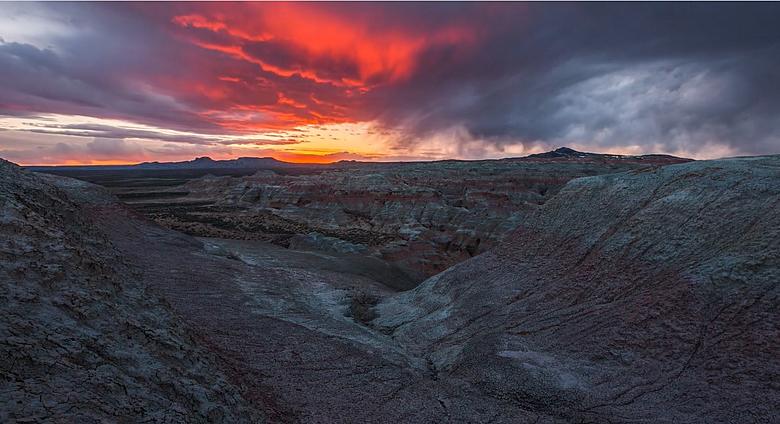This high-angle photograph, captured during sunset in a natural outdoor setting, presents a striking yet desolate landscape. From the vantage point at the top of a mountain, the viewer looks down into a pit-like valley or crater, reminiscent of a volcanic basin. The terrain is predominantly dark gray and stony, devoid of vegetation, further accentuating its barren appearance. 

In the far distance, the landscape extends into a series of plateaus or steps, adding depth and texture to the image. The rocky cliffs exhibit various shades, subtly highlighted by the fading sunlight. The sky above is heavily clouded, casting a backlit glow over the scene that washes out any color, rendering the area in monochromatic hues of gray.

Despite the overcast conditions, the sunset pierces through the clouds, illuminating the sky with a spectrum of reds, oranges, purples, and some pink hues, particularly vivid towards the center. This explosion of colors contrasts sharply with the dark, ominous clouds, suggesting an approaching storm. The interplay of light and shadow, coupled with the dramatic sky, imbues the image with both a raw beauty and a somber, desolate quality.